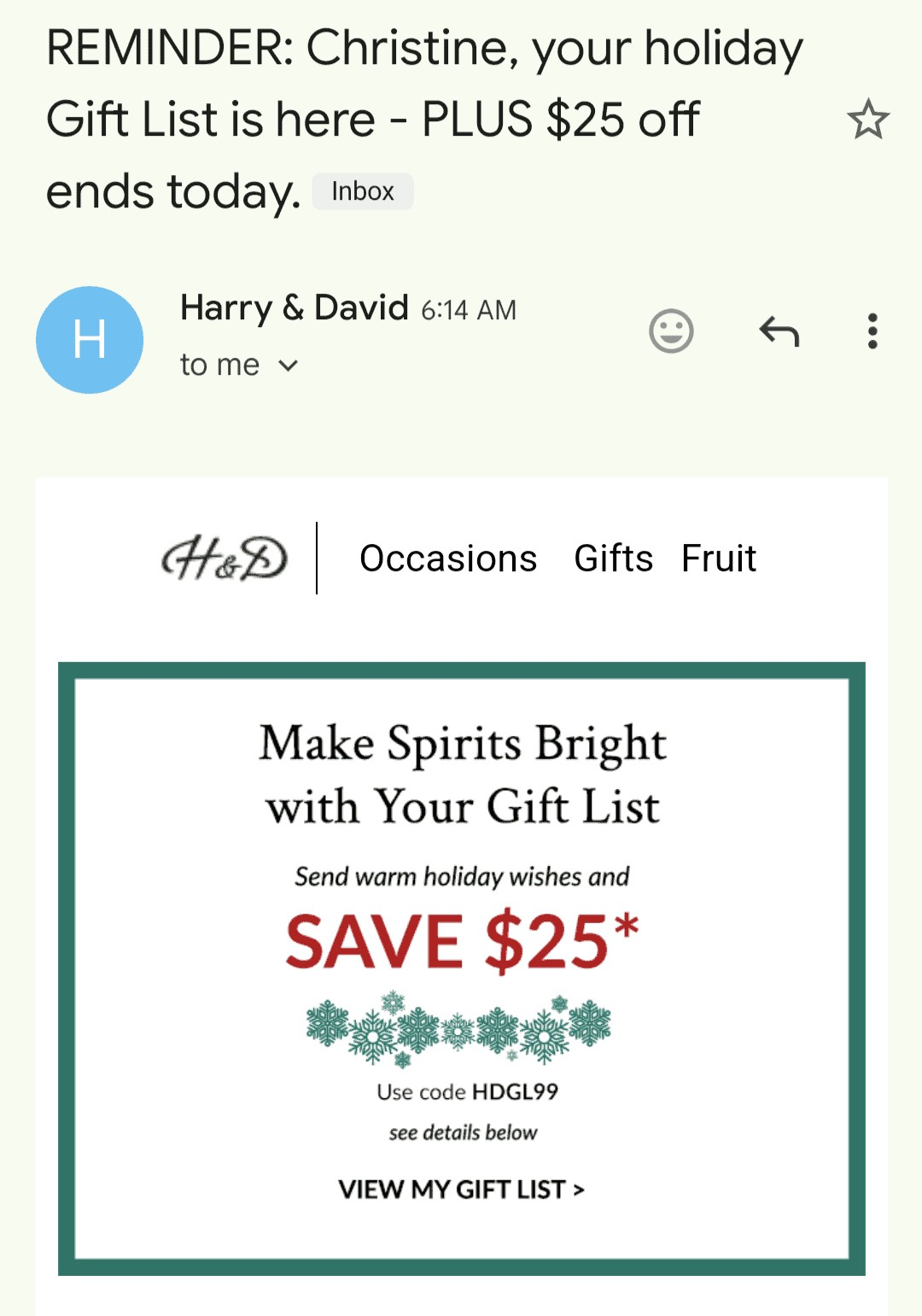The image is a screenshot of a digital reminder from an email, displayed on a cell phone. At the top of the image, there's a banner with a greyish-green background that reads, "Reminder: Christine, your holiday gift list is here – plus $25 off ends today" in white text. Beneath the banner, the word "Inbox" is displayed, indicating the location within the email app.

Immediately below, there's an entry indicating the email is from Harry and David, noted by an 'H' and 'D' logo. The timestamp shows 6:14 a.m., and it's addressed to "me." The Harry and David logo is displayed prominently in ornate letters with the initials "H&D" alongside.

Following the logo, there's a horizontal line separating the header from the main content. The first line of text reads "Occasions | Gift | Fruit," spaced evenly across the screen. Below this, a festive message is shared: "Make spirits bright with your gift list," followed by "Send warm holiday wishes" in a smaller font.

Centrally placed in large, bold red letters is a promotional text that says "Save $25." Beside the "$25," there's a red star for emphasis. Surrounding this promotion are decorative greenish-blue snowflakes.

At the bottom, instructions for redeeming the offer are provided: "Use code HDGL99." There's a note to "see details below" and a button at the very bottom that says "View my gift list."